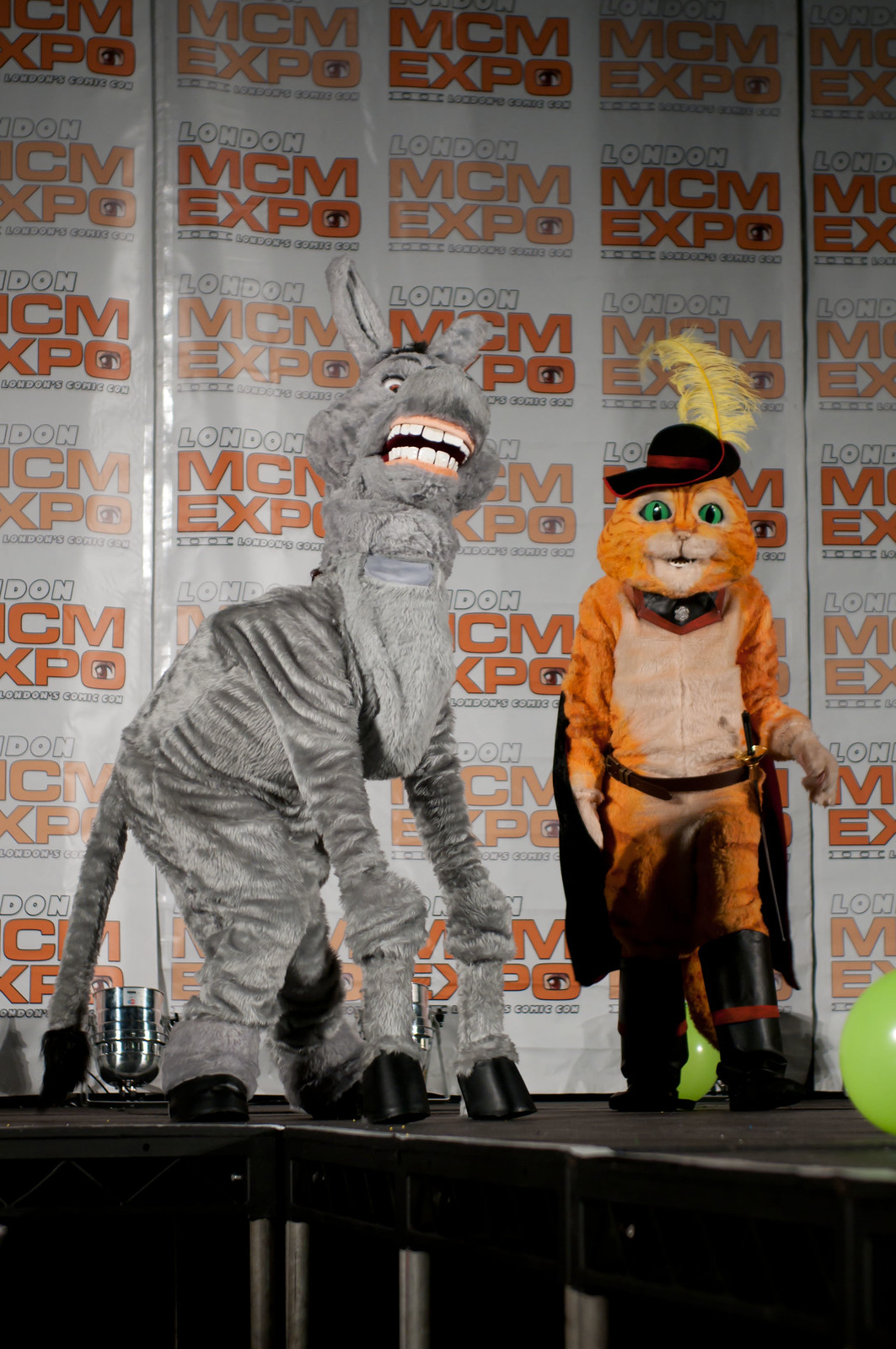In this vibrant photograph from the London MCM Expo, two costumed characters stand prominently on a black stage against a backdrop filled with repeating "London MCM Expo" logos in orange and white. The first character, a large gray donkey, has a big grin and black hooves, with its teeth humorously exposed in classic donkey fashion. Beside it stands an orange feline character, easily identifiable as Puss in Boots, complete with a brown belly, green eyes, black boots, and a distinctive black pirate hat adorned with a yellow feather. Scattered on the stage are a couple of lime-green balloons, adding festive color to the scene. Additionally, there is a silver spotlight near the donkey's tail, casting light upwards. The underbelly of the stage is also visible, contributing to the detailed setting of this lively expo image.